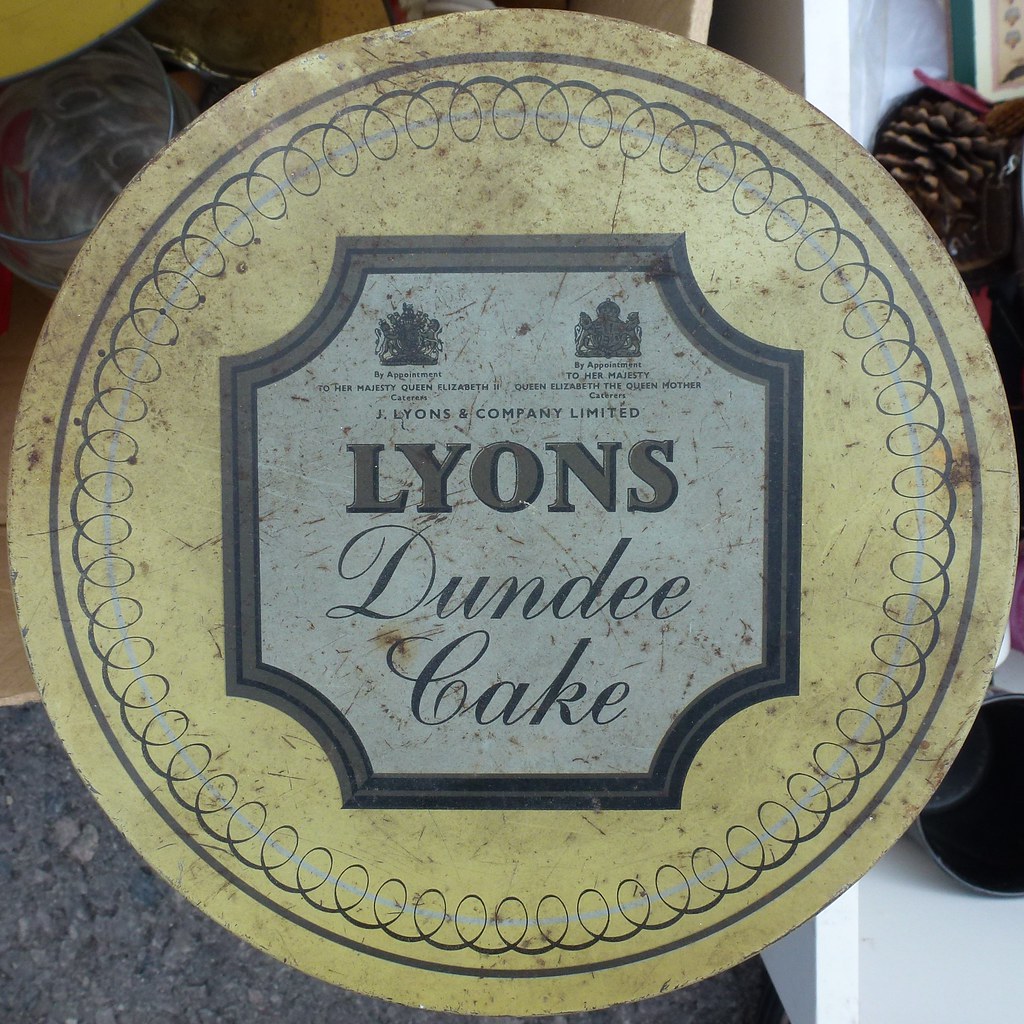The image is a close-up photograph of the top of a very old, antique cake tin, possibly used to store a cake. The lid is an almost dirtied yellow with a weathered, scratched appearance, clearly showing its age and use. There’s a grey border and a repeating grey spiral design on the yellowish background. At the center, there’s a prominent diamond-shaped shield with a white background. Inside the shield, in large grey block letters, it says "J. Lyons and Company Limited," and beneath it, in red script, "Lyons Dundee Cake."

Above this text, the royal insignias and small lettering state, "By appointment to Her Majesty Queen Elizabeth the Queen Mother," signifying its prestigious association with both Queen Elizabeth II and her mother. The tin also features a circular red and white design framing the center shield. The background of the image shows a few kitchen supplies, but the focus remains on this historical cake covering, which appears almost museum-worthy due to its dirt and grime, hinting at its long-lost splendor and rich history.